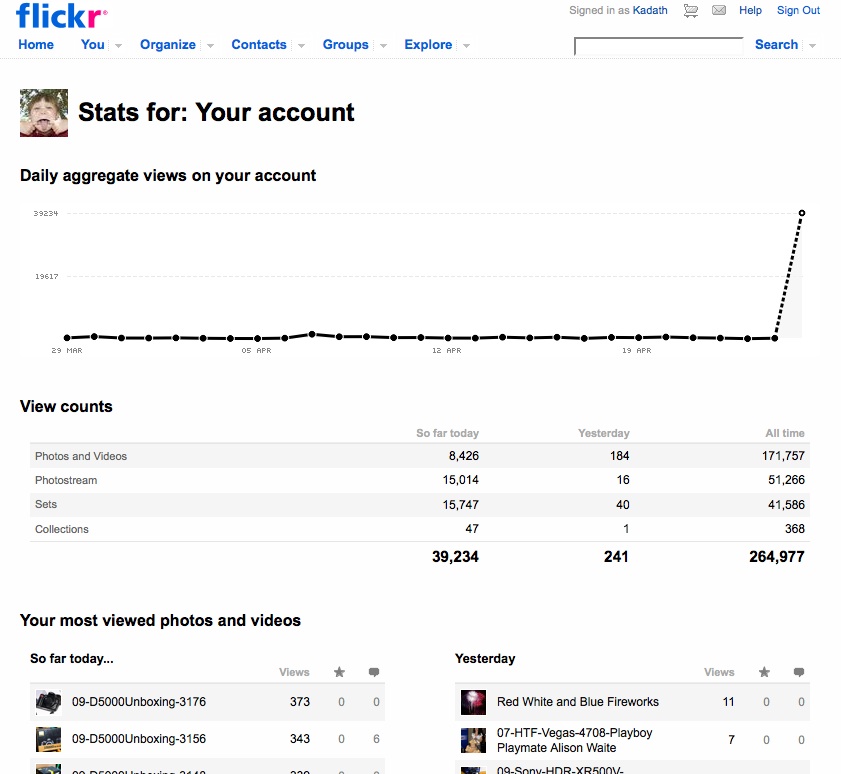The image is a detailed screenshot from the Flickr website displaying user account statistics. In the upper left corner, the Flickr logo is prominently visible; the "Flickr" text is in blue with the "R" in red. Below it are tabs for navigation labeled Home, You, Organize, Contacts, Groups, Explore, and Search, spread across the page. On the upper right, there are icons for a shopping cart, mail, help, and a search bar. It also shows the user signed in as "Kadath" with an option to sign out.

In the upper part of the image, aligned to the left, is a profile picture of a child making a silly face, next to the text "Stats for your account." Below this heading, a section labeled "Daily Aggregate Views on your account" features a line graph, which is mostly flat but spikes at the very end. 

Directly underneath the graph is a detailed table showing view counts. The rows categorize these counts into Photos and Videos, Photo Stream, Sets, and Collections. The columns represent different time frames: So Far Today, Yesterday, and All Time. For example, for Photos and Videos, the counts are 8,426 today, 184 yesterday, and 171,757 all time. 

Following this table, there’s another section titled "Your Most Viewed Photos and Videos." This section includes tables for "So Far Today" and "Yesterday," each listing photo thumbnails with associated view counts, favorites, and comments. Notable entries include a photo titled "09D5000unboxing, 3176" with 373 views, and another titled "Red, white, and blue fireworks" with 11 views. The bottom of the image cuts off additional entries, limiting the visible portion of the statistics.